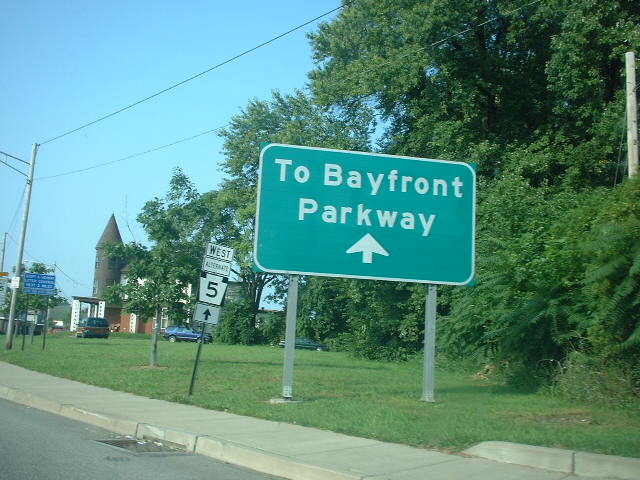This image captures a bustling street bordered by a well-maintained sidewalk and a grassy area. The scene is adorned with various signs and foliage, including several trees and bushes. Prominently featured is a black and white sign indicating directions, where one marker reads "West" and another is partly obscured but might suggest "Alternate." There is also a sign displaying the number "5" with an arrow pointing upwards. A large green directional sign stands out, indicating the way to "Bayfront Parkway" with bold white text and an upward-pointing arrow, all neatly trimmed in white. In the background, a significant structure that appears to be a church or substantial building looms, adding depth to the scene. A few cars are visible, parked on the grassy area, completing the snapshot of this locale.